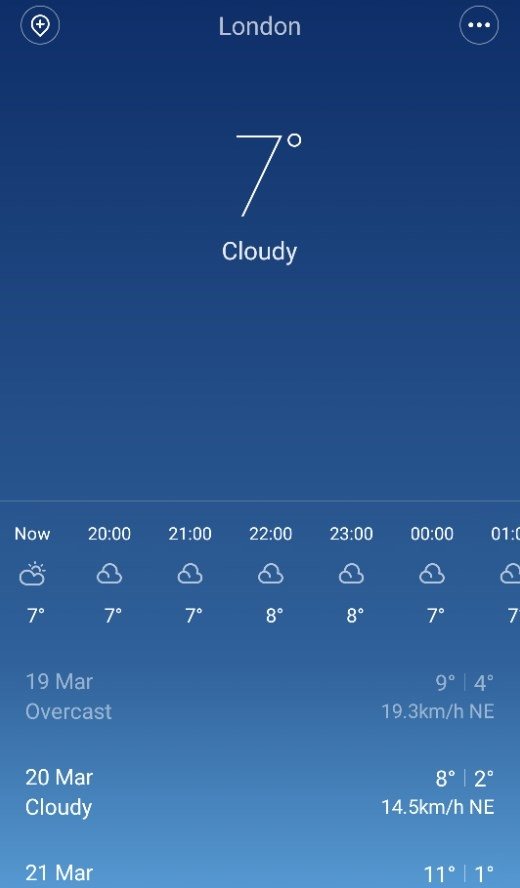This screenshot captures a detailed view of a weather app, featuring a gradient blue background that transitions from a darker blue at the top to a lighter blue at the bottom. The displayed location is "London," prominently shown in the top center of the screen. In the upper left corner, there seems to be an option to add or search for different locations, while the upper right corner features a circle containing three horizontal dots, likely for additional settings or options.

Below the location, the current temperature is displayed as 7 degrees Celsius, accompanied by a "cloudy" weather description. The bottom half of the screen forecasts the weather for the remaining hours of the night, including time intervals at 20:00, 21:00, 22:00, 23:00, and midnight, with temperatures ranging between 7 and 8 degrees Celsius.

Detailed daily forecasts are also provided. For March 19th, the weather is predicted to be overcast with a high of 9 degrees and a low of 4 degrees, accompanied by winds from the northeast at 19.3 kilometers per hour. On March 20th, the forecast indicates cloudy conditions with temperatures peaking at 8 degrees and dipping to 2 degrees, with winds of 14.5 kilometers per hour also coming from the northeast. Finally, the forecast for March 21st shows a high of 11 degrees and a low of 1 degree Celsius.